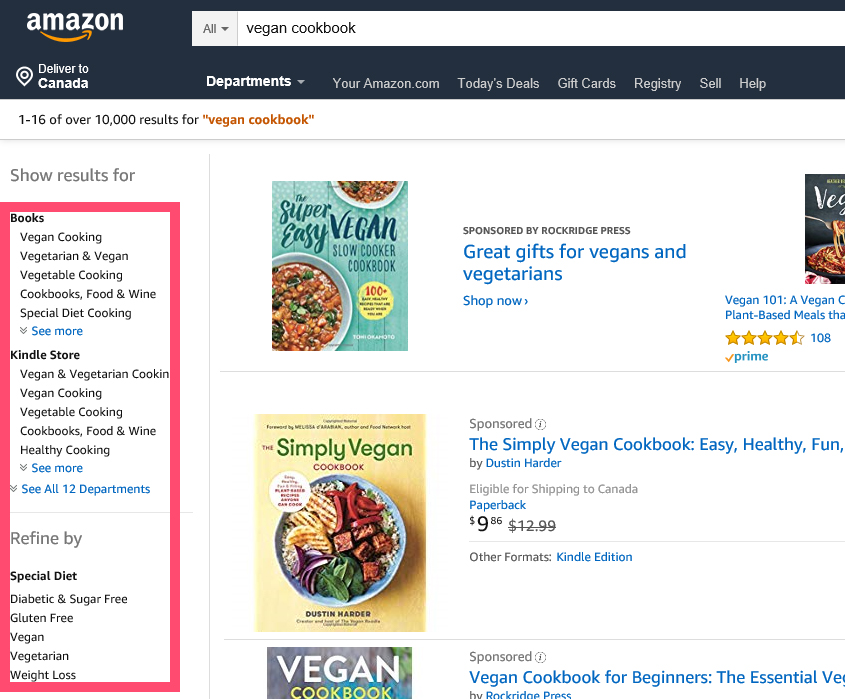This image is a detailed screenshot from the Amazon website. Dominating the top section, a navy blue bar extends across the page, featuring the Amazon logo on the top left. Adjacent to the logo, a search bar with a white background displays the text "vegan cookbook" and indicates that the search encompasses all categories. Below, the website details the shipping location as Canada and offers clickable options for various sections such as "Departments," "YourAmazon.com," "Today's Deals," "Gift Cards," "Registry," "Sell," and "Help."

Following this, a white background displays search results with a header announcing "1 to 16 of over 10,000 results for vegan cookbook," with the term "vegan cookbook" highlighted in bold orange letters. Below this header, individual results are listed:

1. **Sponsored Result by Rockridge Press**: Features "Super Easy Vegan Slow Cooker Cookbook" accompanied by its cover image, suggesting it as a great gift for vegans and vegetarians.
2. **Another Sponsored Result**: "The Simple Vegan Cookbook: Easy, Healthy, Fun" includes the book cover to the left, depicting a bowl of food. Information about pricing, eligibility for shipping to Canada, and availability in various formats such as Kindle edition is also provided.
3. **Vegan Cookbook for Beginners**: Partially visible with the title "The Essential Veg," is listed but gets cut off.

In the left sidebar, users are prompted to refine their search results further by selecting categories such as "Books," "Kindle Store," or narrowing by specific dietary requirements.